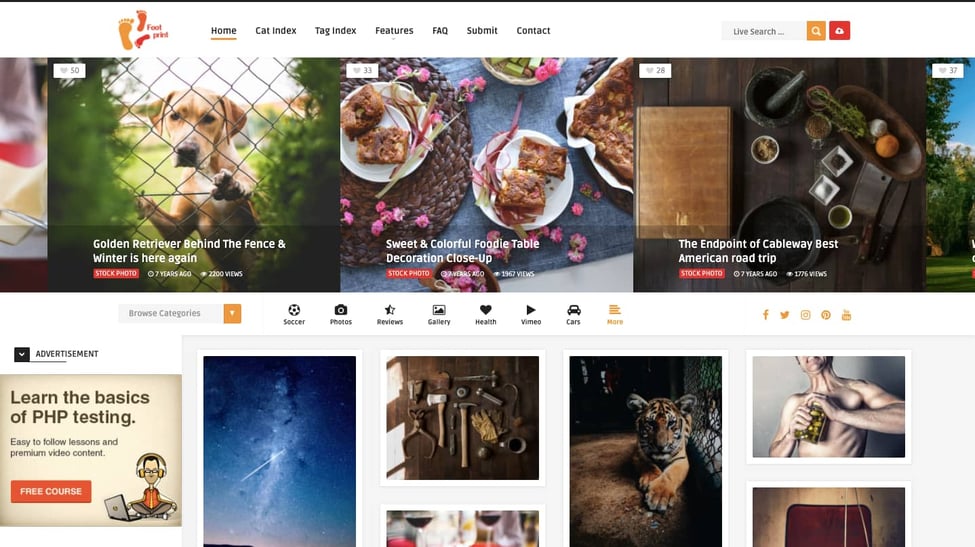Screenshot from the webpage titled "Footprints": the name, written in small font, is located in the upper left-hand corner of the screen. Directly beside it is a graphic containing three orange and red footprints. The top navigation bar displays tabs labeled Home, Cat Index, Tag Index, Features, Back, Submit, and Contact, along with a search bar reading "Live Search."

Below the navigation bar are three distinct images. The first image shows a golden retriever puppy behind a fence, captioned “Golden Retriever Behind the Fence, Winter is Here Again.” Despite the caption indicating winter, the photograph showcases lush greenery. This image is tagged as a stock photo, noted in a red bar, and is dated seven years ago. It has garnered 2,200 views and received 50 hearts.

Next to it, there is an image of an assortment of food titled “Sweet and Colorful Foodie Table, Decoration, Close Up.” The image, also designated as a stock photo within a green rectangle, is difficult to date due to slightly blurry white text but is estimated to be from seven years ago. The photo features a loaf dish placed on a white plate adorned with flowers and has accumulated 1,967 views.